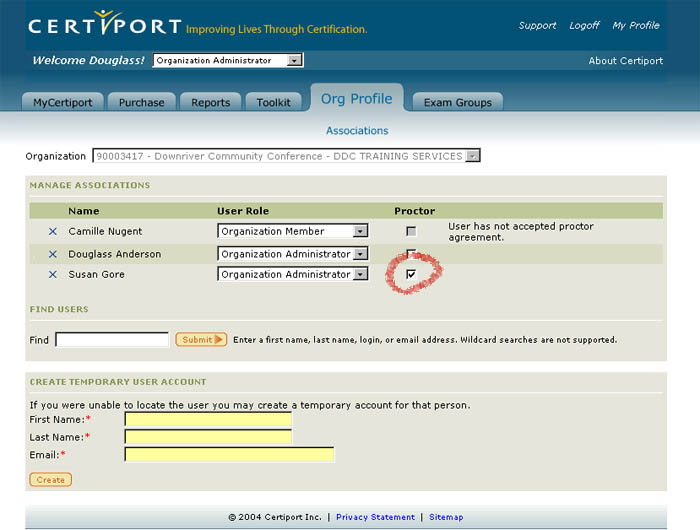Screenshot of CertiPort Website Interface:

The screenshot captures the interface of the CertiPort website, clearly designed for administrative management. In the top left corner, the CertiPort logo is prominently displayed with the tagline "Improving Lives Through Certification." On the top right, links for "Support", "Log Off", and access to "My Profile" are visible.

Immediately beneath this header is a welcome message for the user, "Welcome, Douglas", accompanied by a dropdown menu indicating the user's role as "Organization Administrator." The interface features several navigational tabs, with the "Org Profile" tab currently active.

Further down, the selected organization is "Downriver Community Conference (DCC) Training Services," and the section heading is "Manage Org Associations." The interface is organized into columns labeled "Name", "User Role", and "Proctor." The first entry is "Kamel Nugent", identified as an "Organization Member", with a note stating "User has not accepted proctor agreement." The subsequent entries are "Douglas Anderson" and "Susan Gore", both listed as "Organization Administrators." Notably, there is a checkbox next to Susan Gore's name, marked and encircled in red.

Below the user list, a "Find Users" section with an empty search box and a "Submit" button is located. Further down, there is an option for creating temporary user accounts, complete with fields for "First Name", "Last Name", and "Email", all accompanied by blank text boxes. At the bottom of this section is a "Create" button.

The interface is designed to facilitate user management within the CertiPort certification platform, providing various tools for administrators to oversee and modify user access and roles efficiently.